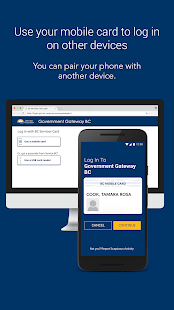This image is a vertically-oriented screenshot with a solid dark blue background. At the top, white text reads, "Use your mobile card to log in on other devices." Below this, in smaller centered white text, it says, "You can pair your phone with another device." The center of the image features an illustration of a computer monitor with a black border and a silver base. The screen of the monitor is on, displaying a white background with a blue banner across the top. To the lower right of the monitor is an illustration of a black cell phone showing a white screen. Although the text on the phone is blurry, it appears to display the name of a user.